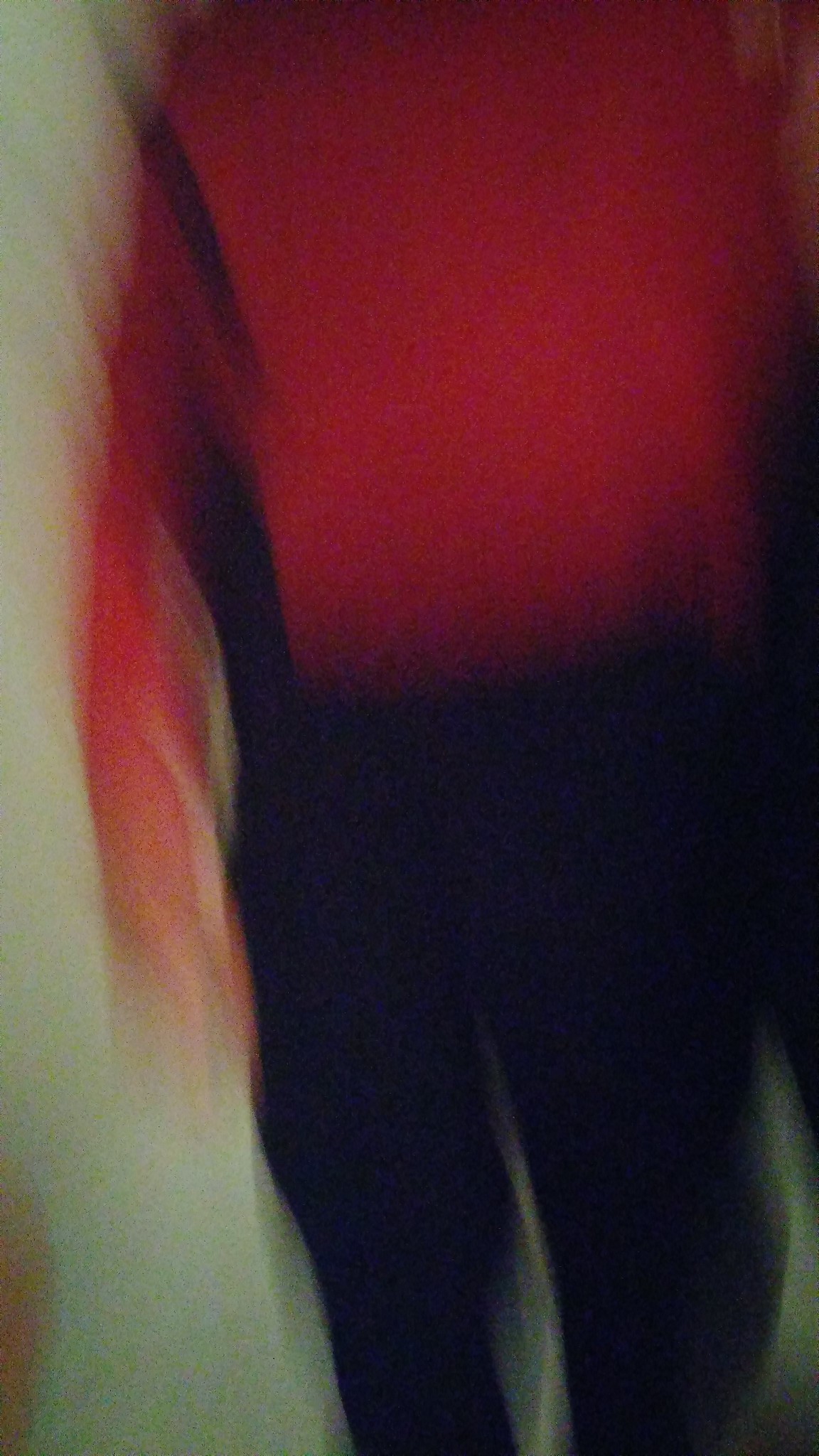The photograph features a tall individual dressed in black pants and a red long-sleeve shirt, standing in front of a heavily blurred white wall. The person's head is not visible in the frame, but the torso and the right arm are clearly shown. The right arm, positioned on the left side of the image, has noticeable shadows near the bicep and underneath the arm. In the bottom left corner of the photograph, there is a small brown object, although its exact nature is indiscernible. The overall color contrast between the person's attire and the softly diffused background makes the subject stand out in the image.